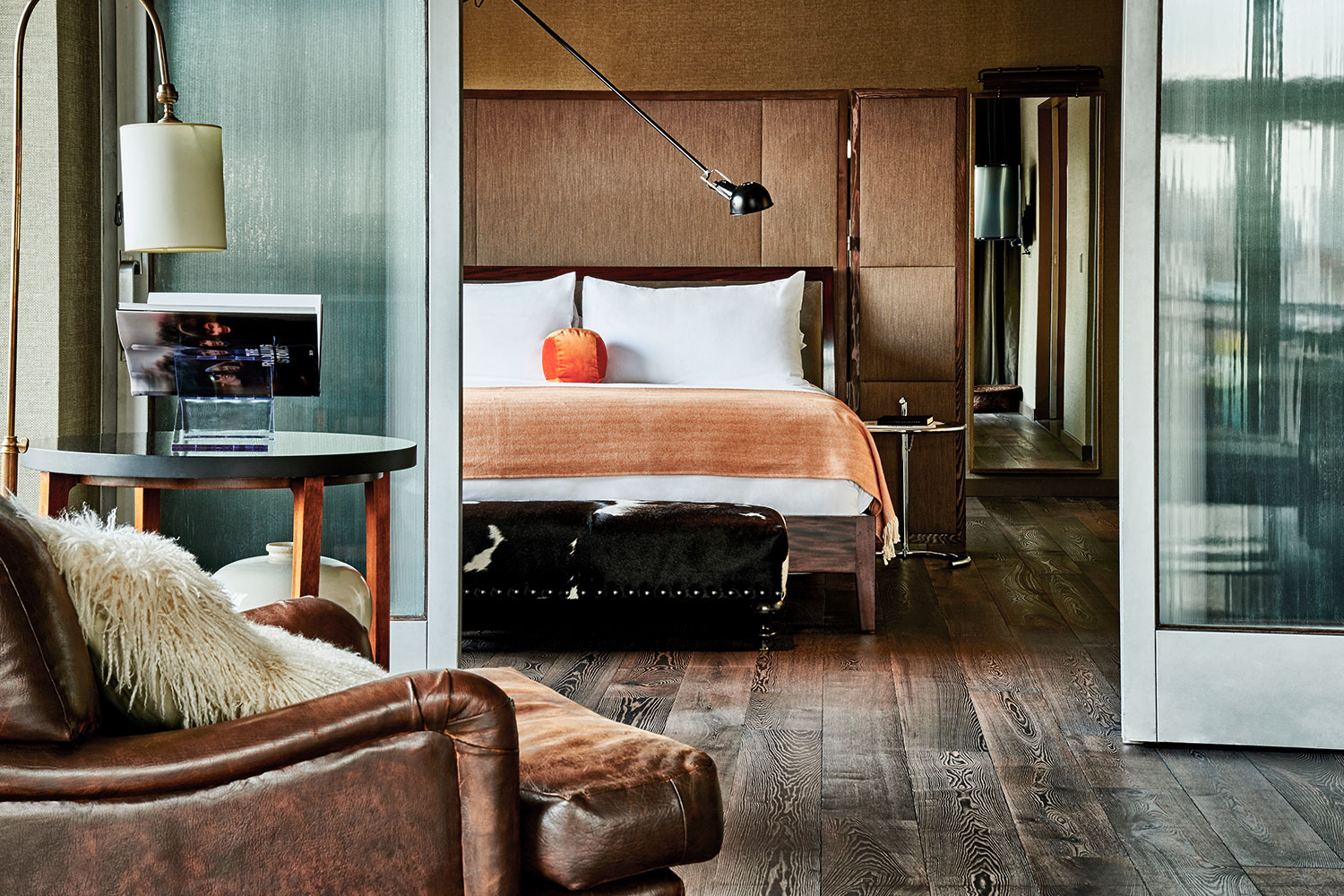This photograph, taken from the living room, offers a detailed look into a distant bedroom. The living room features dark brown wooden floors made of rectangular planks. In the bottom left corner is a cozy light brown leather armchair adorned with a white Chanel pillow. Next to the armchair is a round table with a black surface and four light brown legs, topped by a white acrylic stand holding an open book. A bronzed floor lamp arches over the table, casting light directly onto it. On the floor beneath the table rests a large, bulbous white porcelain vase with a tiny top opening.

The living room opens to the bedroom through a set of glass doors. Inside the bedroom, which is designed to accommodate two people, there's a bed with white pillows. At the foot of the bed sits a small leather couch without a back, potentially serving as a storage bench. To the right of the image near the bed is a small book stand, and another door leads into a separate room. A window on the left side of the image frames a view of the cozy chair in the foreground. The overall scene creates a harmonious blend of comfort and style, with carefully curated furnishings and thoughtful decor.